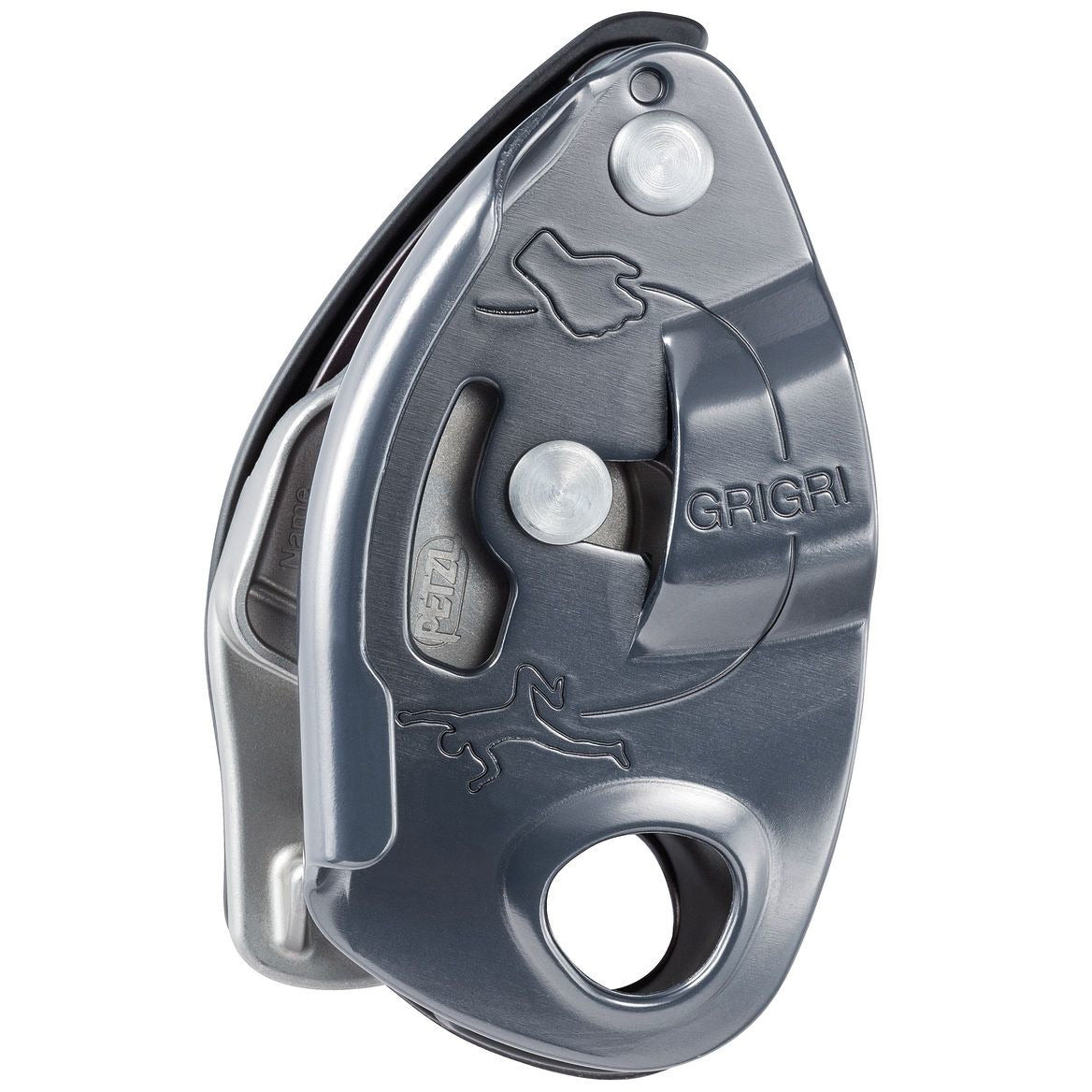The image is a color, portrait-oriented photograph of a silver, metallic foldable tool that has an elliptical, egg-like shape—narrow at the top and wider at the bottom. The top portion of the tool is attached with a round silver screw and features a mechanism on the left side that appears to be a pop-out knife. The tool prominently displays the word "GRIGRI" in capitalized letters at its center.

The surface of this tool includes a detailed illustration. On the top half, an image is embedded, depicting the outline of a man with his left foot lifted, connected by an arrow to a right hand that seems to be holding a rope or curved object. This design suggests it might be related to climbing or hiking equipment, possibly a carabiner. The illustration wraps around, leading to an additional outline that seems to show a person either running away or lying down, adding to its utilitarian and potentially safety-related imagery. The overall photographic style is representational and realistic, focusing on product photography.